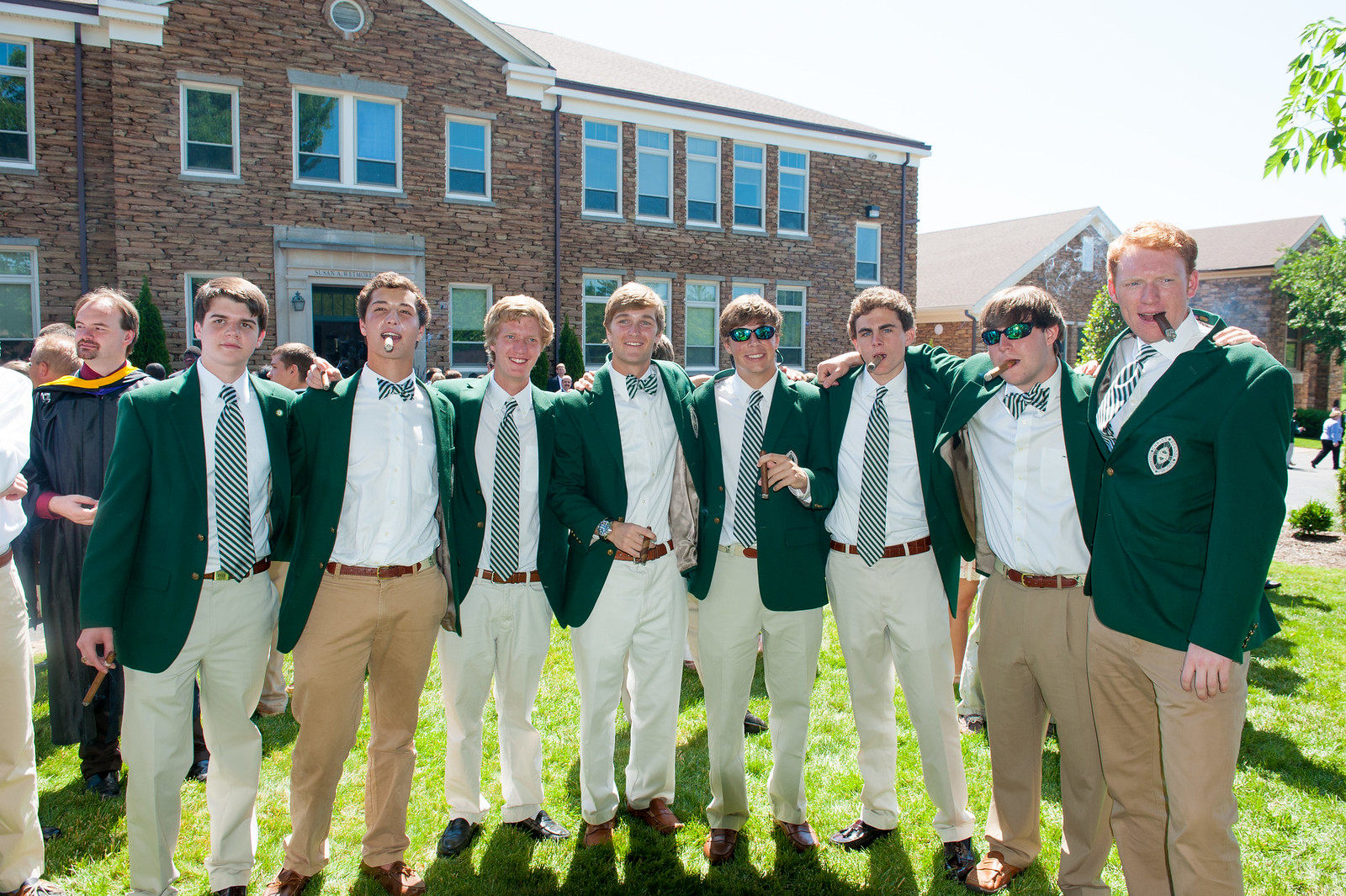In this bright and sunny photograph, a group of eight young men, likely college students part of a fraternity, stand arm-in-arm on a lush green lawn. They are dressed uniformly in dark green blazers over long-sleeved white collared shirts, with matching green and white striped ties, some opting for neckties while others display bow ties. Their light khaki or whitish pants, brown belts, and occasional sunglasses add to their coordinated attire. Many of them hold cigars, and a few are smoking them, suggesting a celebratory occasion. The group stands in front of a large, gray brick building, possibly a dormitory, characterized by several windows and a prominent arched doorway at its center. The clear shadows cast in front of them underline the bright, sunny day. In the background, additional people and even a glimpse of a graduation gown are visible, adding to the festive atmosphere. The men all smile at the camera, capturing the joyous spirit of the moment.